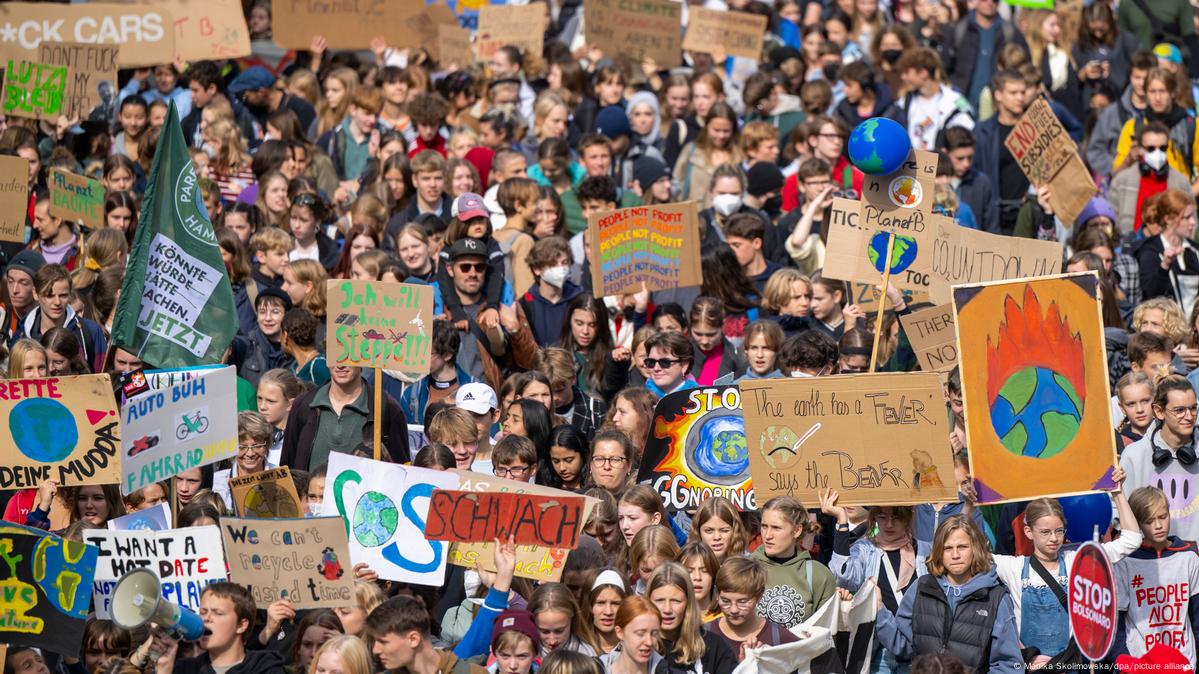The image captures a densely packed crowd of environmental protesters, pressed together like sardines, in a horizontal, landscape-mode color photograph taken outdoors from a slightly elevated angle. Predominantly composed of pale-skinned individuals, the crowd is vibrant with an array of brightly colored, mostly cardboard signs in multiple languages, including English, German, and Spanish, reflecting a global movement. Key messages on the posters include "Stop Ignoring," a painted depiction of the Earth engulfed in flames, "The Earth has a Fever" accompanied by a bear illustration, and another repeated slogan "People, not Profit" in rainbow colors. Among the sea of signs, one protester in the lower left corner wields a blue and white megaphone, adding to the dynamic atmosphere filled with shouting and chanting.